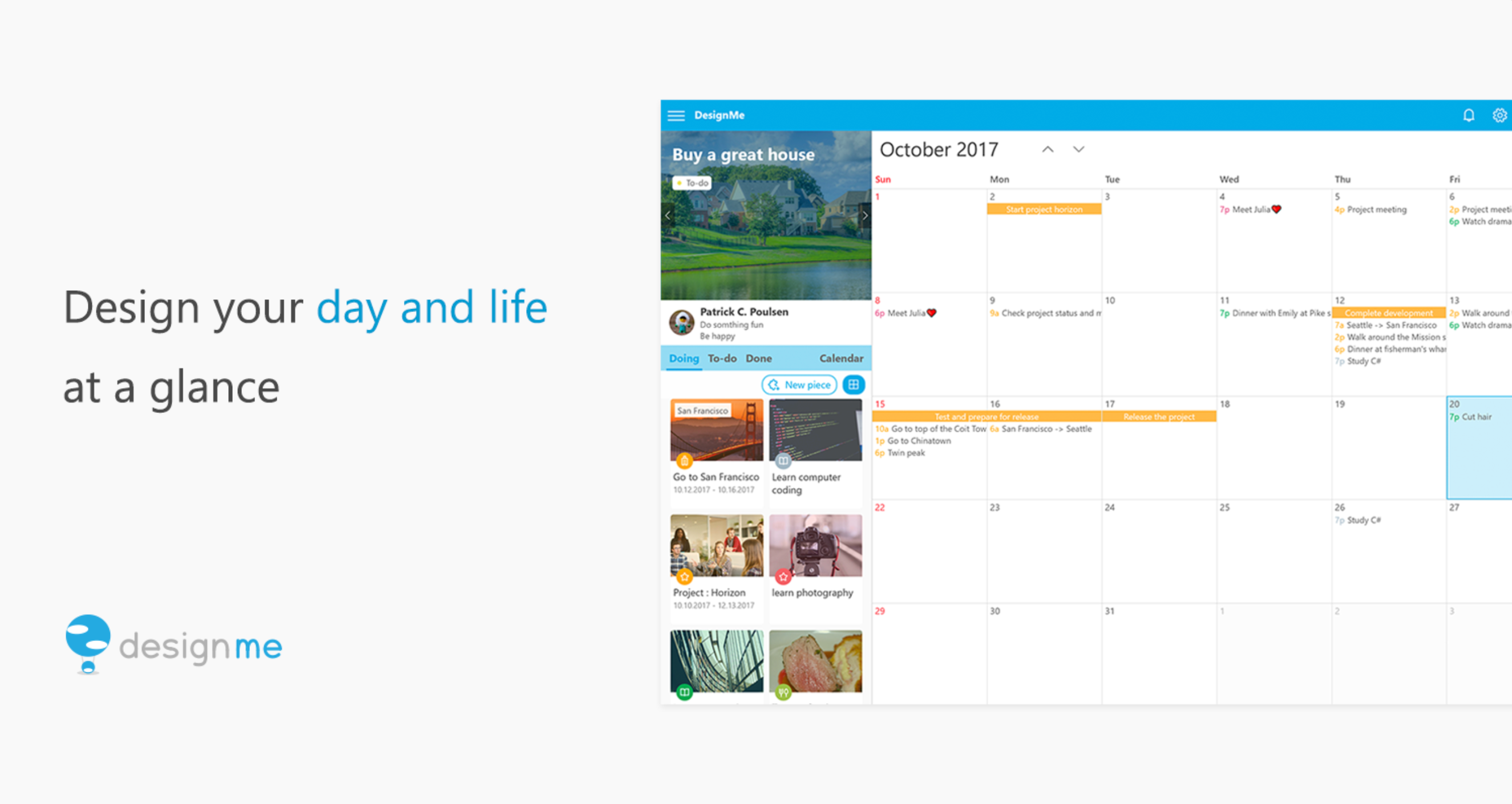The image displays a screenshot of a web page, specifically the main landing page of a site named "Design Me." The backdrop of this page is a plain light gray, which also forms the outer border of the screenshot. Dominating the left side of the image is large text in gray and blue that reads, "Design your day and life at a glance." Above this text, there is a stylized logo featuring two blue dots: one large dot with two white ovals positioned in the center, and a smaller dot beneath it with a single white oval in the center. 

At the top of the web page, there's a bright blue border. On the left side within this border, a hamburger menu icon is visible, followed by white text that says "Design Me." On the right side of the blue border, there are two additional white icons - one depicting a bell and the other a gear, likely indicating notifications and settings, respectively.

On the left side of the main web page, a column of small thumbnail photos is displayed. Each thumbnail has a multicolored icon superimposed on its bottom left corner. The first photo is labeled "San Francisco" with a white label featuring black text, and underneath it, black text reads "Go to San Francisco." Following this, other photos are similarly labeled: "Learn computer coding," "Project Horizon," and "Learn photography."

The central body of the web page showcases a calendar interface. At the top of this calendar, the days of the week are listed abbreviated as "Sun, Mon, Tue, Wed, Thu, and Fri." Above these abbreviations, bolded text reads "October 2017," flanked by up and down arrows, presumably to navigate through different months. Each calendar date box, numbered from 1 to 31, contains various entries. Some dates feature small yellow banners with white text, with tasks such as "Start Project Horizon," "Complete Development," "Release the Project," and "Test and Prepare for Release." Other dates include personal engagements, such as "Meet Julia" with a bright red heart icon, "Project Meeting," "Watch Drama," "Dinner with Emily," "Walk Around," "Check Product," and "Project Status," alongside tasks like "Study."

The screenshot provides a thorough overview of the "Design Me" web page layout, illustrating its functionality designed for organizing both personal and professional activities.